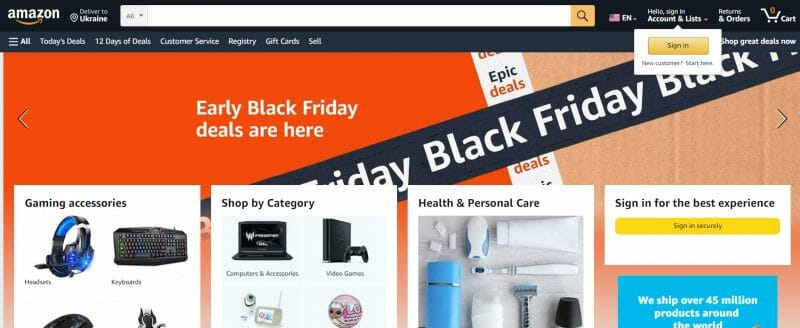This image is a screenshot of the Amazon website. In the upper left corner, the Amazon logo is prominently displayed along with a notification indicating that delivery is available to Ukraine. At the top center of the webpage, a search bar is visible, set against a navigation bar where the language preference is set to English. To the right of the search bar, there are options for signing in, viewing returns and orders, and an indication that the shopping cart is currently empty.

Directly beneath this navigation bar, a series of tabs are visible, including options for "All," "Today's Deals," "12 Days of Deals," "Customer Service," "Registry," "Gift Cards," and "Sale." Below these tabs, an eye-catching orange banner stretches across the width of the page. On the right side of this banner, an image of a cardboard box is featured, adorned with "Black Friday" and "Epic Deals" labels. The text on the orange portion of the banner reads, "Early Black Friday deals are here."

Further down the webpage, there are three distinct sections. On the left, there is a category labeled "Game Accessories." In the center, the site offers a "Shop by Category" section. On the right side, there is a section for "Health & Personal Care" along with an additional sign-in prompt.